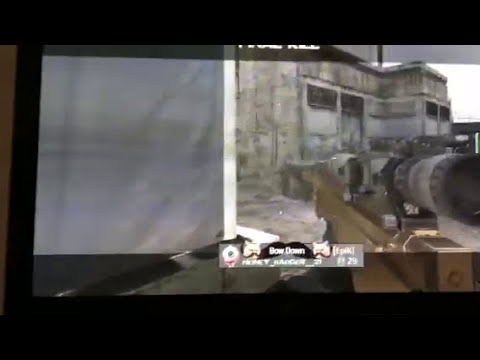The image is a screenshot from a video game, specifically a first-person shooter. Dominated by gray, tan, and white hues, the scene captures the player’s perspective holding a goldish sniper rifle with a black and white scope. At the bottom of the image, text reads "bow down," accompanied by an animated mustache flanked by cats, with the word "honey" visible beneath one of the cats, which could denote a screen name. To the left, a featureless gray blur shares the space, while the right side showcases an old stone or cement building with windows, suggestive of an aged structure. The building appears somewhat blurred, complicating visual clarity. The player points the weapon at a series of doors and lacks visibility of any targets or characters in sight.